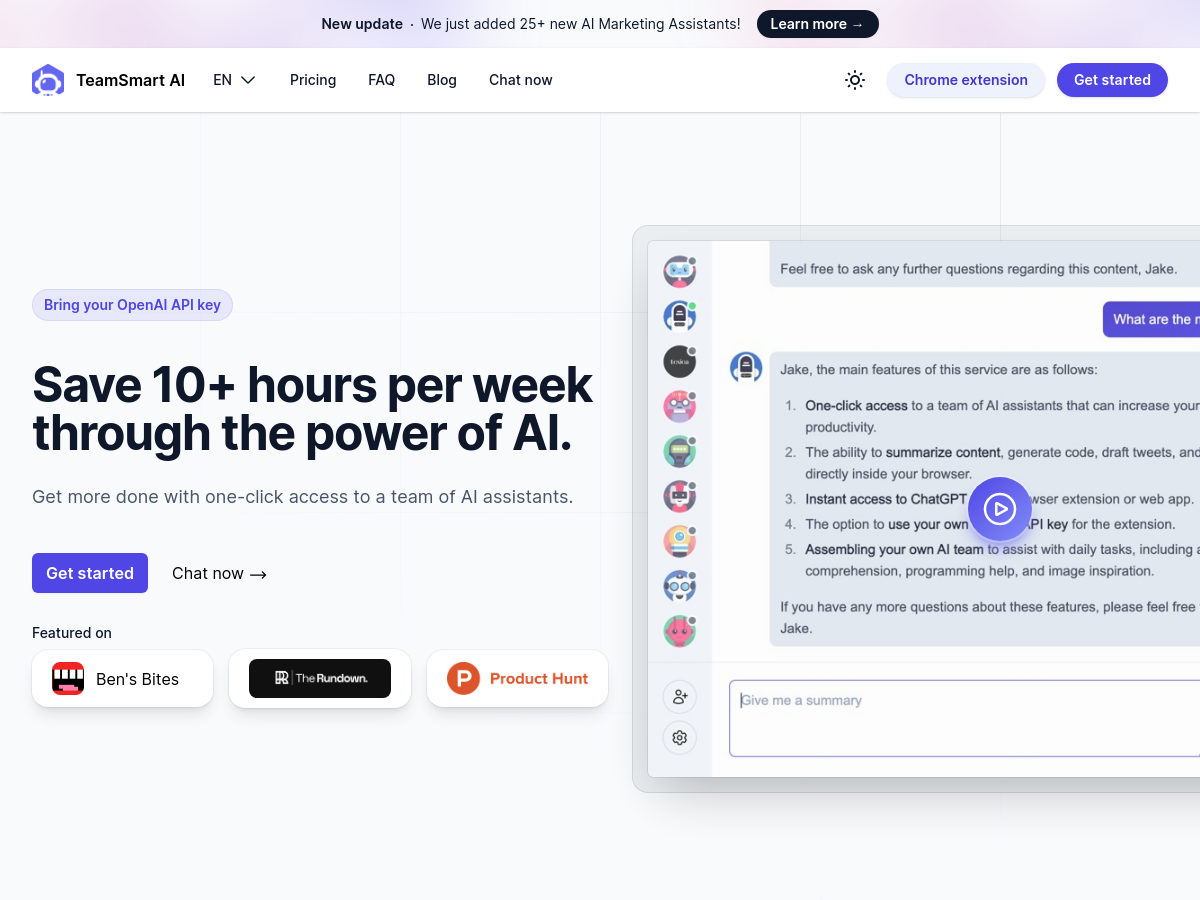This is a detailed screenshot of a website that appears to be an advertisement. At the top, there's a light blue banner with the text "New Update: We just added 25+ new AI marketing assistants" displayed in black font. Beside this text, there's a small black oval with "Learn More" written in white font accompanied by a downward arrow, indicating a dropdown menu.

Below the banner, there is a white rectangular section featuring the title "Team Smart AI." This section includes an icon of an astronaut head in white on a blue diamond background. To the right, there's a language selection option indicating English has been chosen. Adjacent to that are navigation links labeled "Pricing," "FAQs," "Blog," and "Chat Now."

Further along, there is a blue-and-white oval button with "Chrome Extension" written in blue font. Next to it is a dark blue oval button stating "Get Started" in white font.

The main body of the ad reads: "Bring your OpenAI API key, save 10+ hours per week through the power of AI, get more done with one-click access to a team of AI assistants." Below this, there's a small blue rectangle with "Get Started" written in white font. Beside it, in black font, it says "Chat Now" with a right-pointing arrow.

At the bottom, it notes that the service is featured on "Ben's Bites" and "Product Hunt."